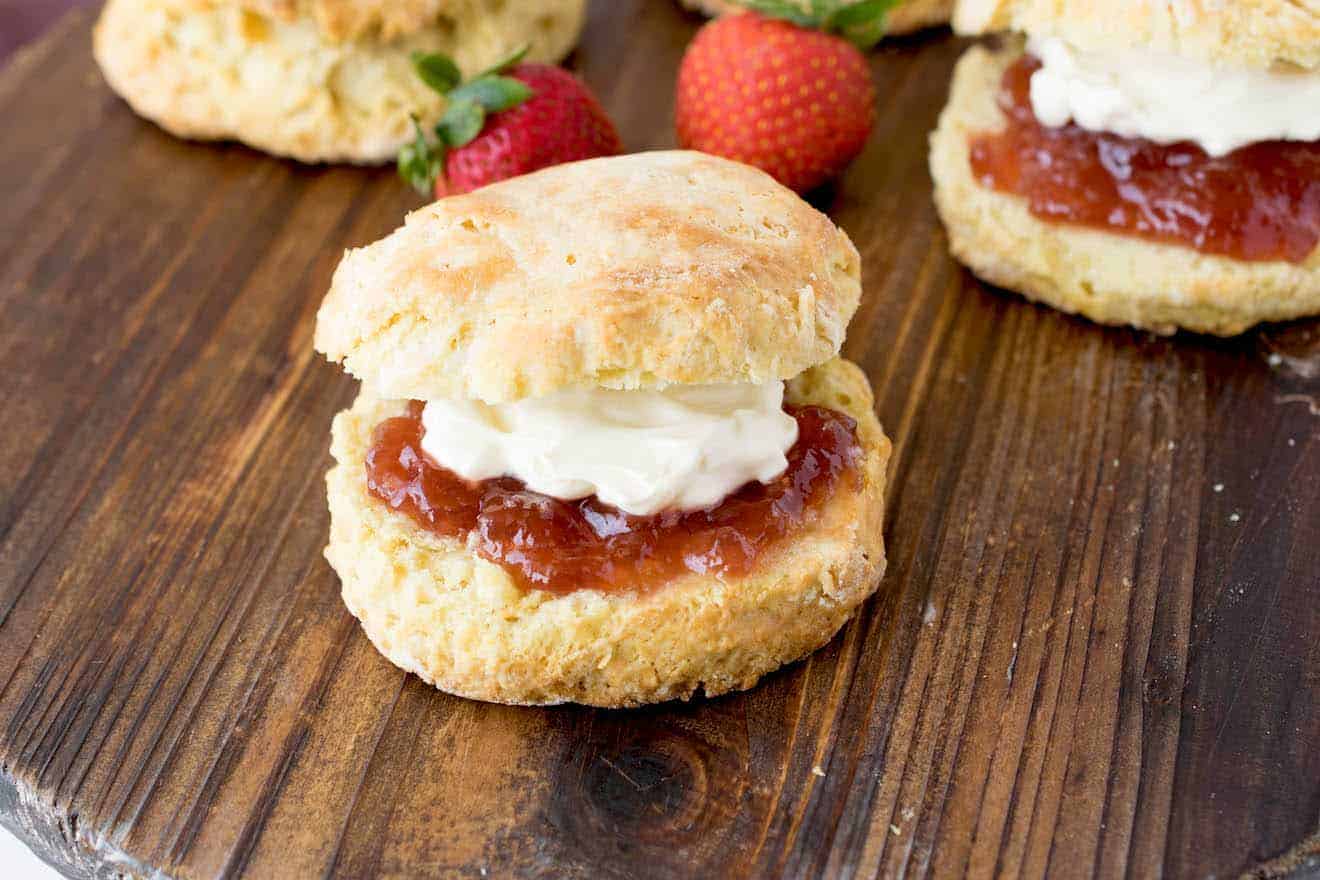In the image, there are three English muffins arranged on a dark wooden surface that could be a table or a cutting board. At the center, two strawberries accompany a fully assembled English muffin sandwich filled with a reddish strawberry jam and topped with a white, swirled cream cheese. To the right, a similarly prepared English muffin is visible, while on the left, a whole English muffin remains uncut and unfilled. The muffins appear homemade, evident from their uneven sizes and fluffy texture. The color palette is dominated by the browns and tans of the muffins, contrasted by the vivid red of the strawberry jam and bright white of the cream cheese.